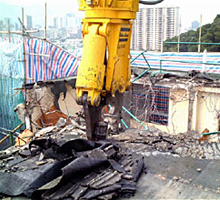The photograph captures the demolition of a building, featuring a large, yellow demolition tractor with a black-tipped claw actively tearing through the structure. The building, a single-story white-walled construction, is in ruins with debris and rubble scattered around the lot. A blue, white, and green striped tarp, part of which is falling, serves as a partial railing on the roof. Black tarps and makeshift wooden railings are visible in the scene, likely used for temporary safety measures. Tall green trees and distant city buildings, including a strikingly high residential high-rise and a white building reminiscent of a hotel, frame the background under an overcast sky. The scene is illuminated by natural, diffused daylight, emphasizing the ongoing chaos and the texture of the pared-down building materials.